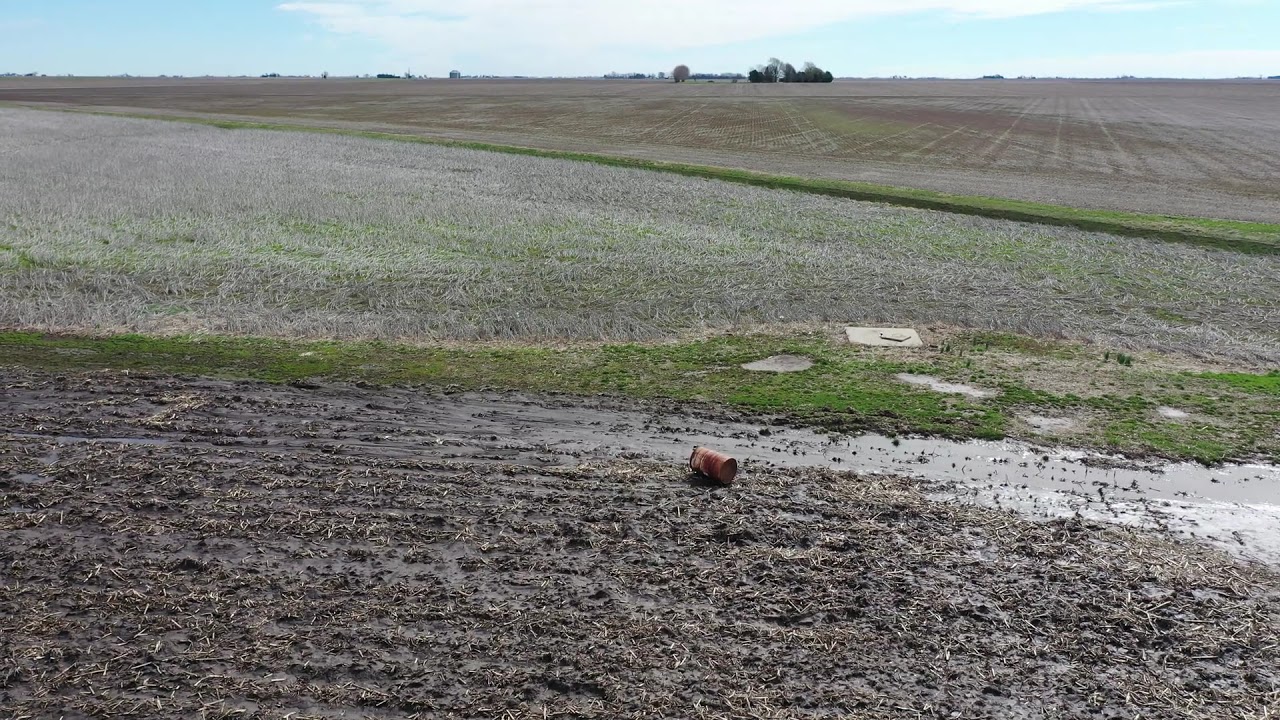In this image of a desolate farmland, the foreground features a strip of severely beaten grass and patches of dried, wet mud. The ground is marred by three indentations, one square and two round, indicative of heavy machinery activity. At the center, a rusted tin can lies amid worn soil so compacted and eroded that it forms small puddles. A piece of trash is also discernible in the scene. Further into the image, the farmland appears slightly more structured with a pattern suggesting recent tilling for crop growth. In the far distance, small structures or homes and possibly some trees are visible against a clear blue sky, marking the boundary of this rugged landscape. The overall condition of the dirt and grass suggests intense wear, raising doubts about its viability for future cultivation.